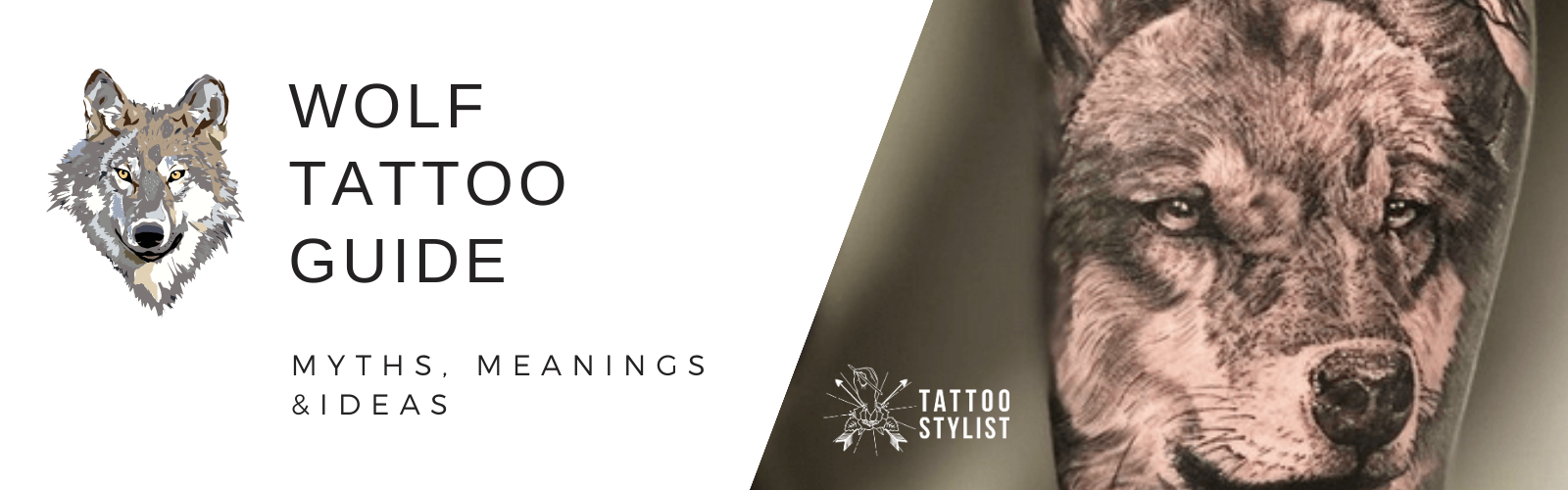The image is a digital poster promoting a product or brand related to wolf tattoos. The left side of the poster features an illustration of a wolf facing the camera, set against a white background. To the right of this illustration, bold black text reads "Wolf Tattoo Guide," and directly below it, in smaller text, "Myths, Meanings, and Ideas." The right side of the poster showcases a close-up black-and-white tattoo of a wolf's face on a body part, with the exact location being ambiguous, possibly an arm or a thigh. This side has a muted grayish-green background, adding depth to the composition. At the bottom left of the tattoo image, the text "Tattoo Stylist" appears in white, accompanied by a logo featuring two arrows pointing outward from a central, indistinguishable element encircled by radiating lines, resembling a starburst pattern. The overall background is slightly blurred to emphasize the detailed wolf tattoo.